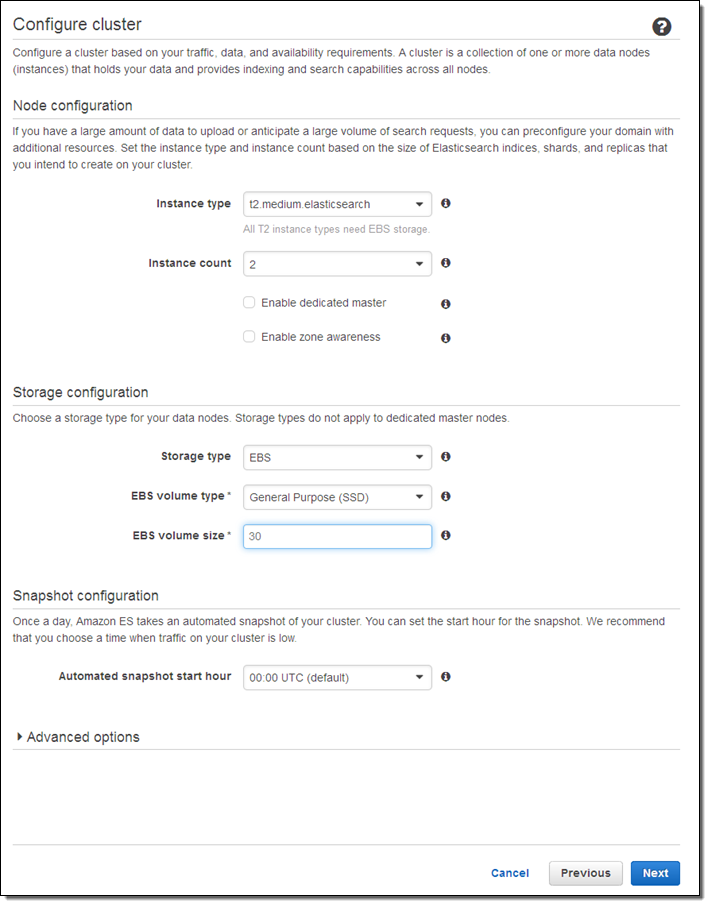The screenshot depicts a white page from a configuration interface. In the upper right-hand corner, there is a question mark icon. The first prominent header reads "Configure Cluster". This section allows users to set up a cluster based on their traffic data and additional parameters. 

Below this header, there is a "Node Configuration" section where users can select and modify the instance type and instance count.

Following that, there is a "Storage Configuration" section. Here, users can adjust the storage type, specify the Amazon EBS (Elastic Block Store) volume type, and determine the EBS volume size.

The next section is "Snapshot Configuration," which enables users to set the automated snapshot start hour. The current setting is 00:00 UTC, which is the default.

Lastly, there is a "Advanced Options" heading. 

In the lower right-hand corner of the page, there are three navigation options: a "Cancel" link, a "Previous" link, and a "Next" button highlighted in blue.